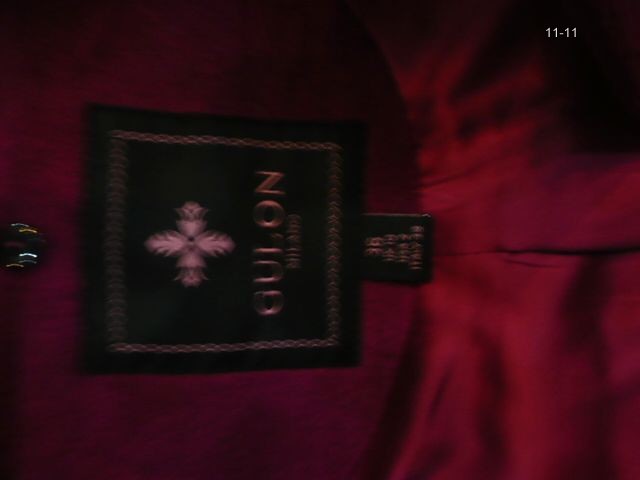This extremely blurry, sideways close-up photo captures a tag from an article of clothing, which is aligned with the right side as the bottom. The tag displays a black square with a plus-shaped white emblem or leaf pattern at the top and the letters G-U-L-O-N, believed to be gold-colored, prominently below. The black square tag is bordered by a decorative gold edge. Below the main tag is a smaller, attached tag with size information, noted as "36," but further details are indiscernible due to the blurriness. The plush-looking red fabric with a sheen provides a striking background. In the top right corner of the image, the watermark "11-11" is clearly visible.